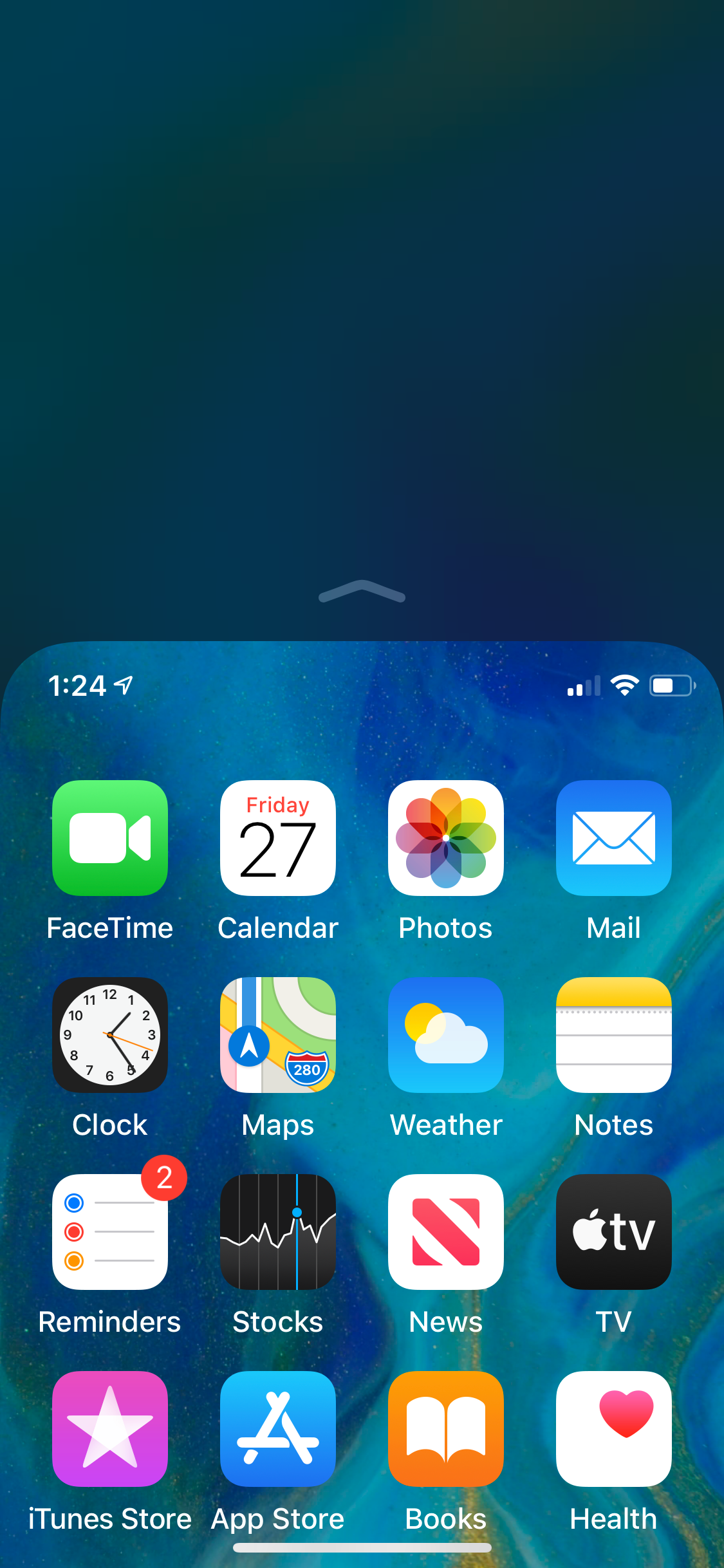The image depicts a digital interface with a dark navy blue background at the top, transitioning to a lighter blue color towards the bottom. At the midpoint of the image, an upward-pointing arrow is present. Below the arrow, the screen displays the number "124," along with two signal bars and a half-full battery icon. The interface is populated with four rows of four app icons, each labeled with its respective functionality.

- **Top Row:**
  - **Top Left:** A green box with a camera icon labeled "FaceTime."
  - **Second from Left:** A white box with the date "Friday 27th" labeled "Calendar."
  - **Third from Left:** A multi-colored flower icon labeled "Photos."
  - **Top Right:** A blue box with an envelope icon labeled "Mail."

- **Second Row:**
  - **First on the Left:** A black box with a clock icon labeled "Clock."
  - **Second from Left:** A map icon labeled "Maps."
  - **Third from Left:** An icon depicting a blue sky with a cloud and sun, labeled "Weather."

The described interface likely belongs to a smartphone or tablet, showcasing a typical home screen layout with essential apps and status indicators.